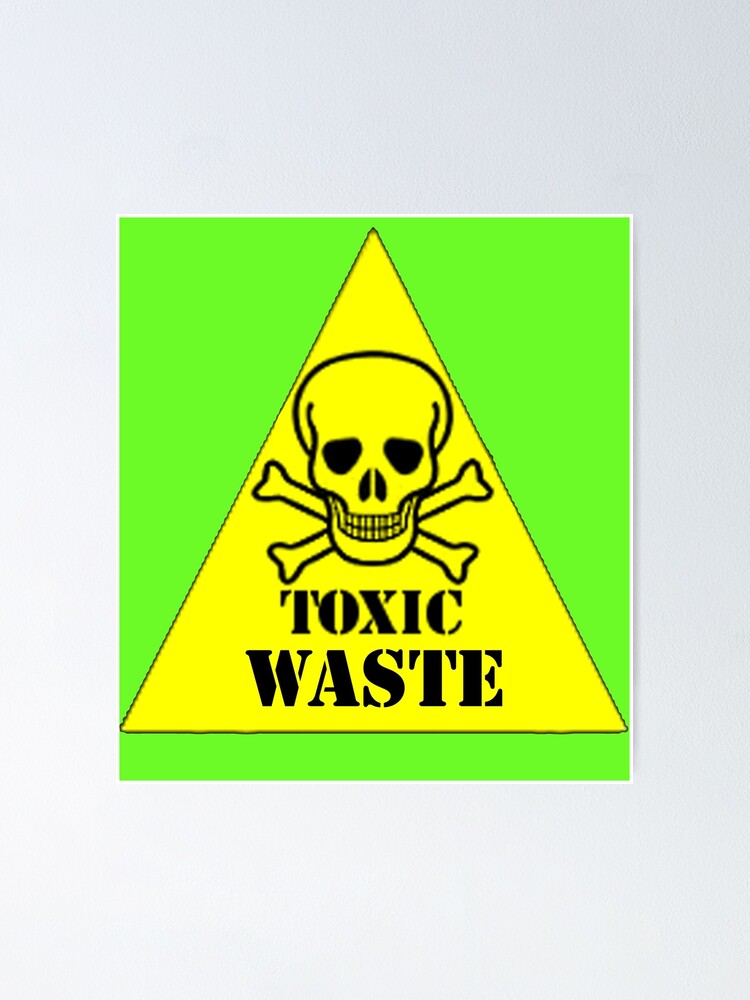The image showcases a vertically oriented rectangular sign set against a light gray wall. At the center of this sign is a neon green square background with a thin white border. Dominating the neon green square is a large yellow triangle. Inside the triangle, at the top, is a black-outlined skull with detailed crossbones extending behind it. The eyes and the nose of the skull are filled in solid black. Beneath this ominous symbol, the words "TOXIC WASTE" are prominently displayed in bold, black, all-caps letters, centered one on top of the other. The overall design uses vivid colors and stark contrasts to create a striking and attention-grabbing warning sign.